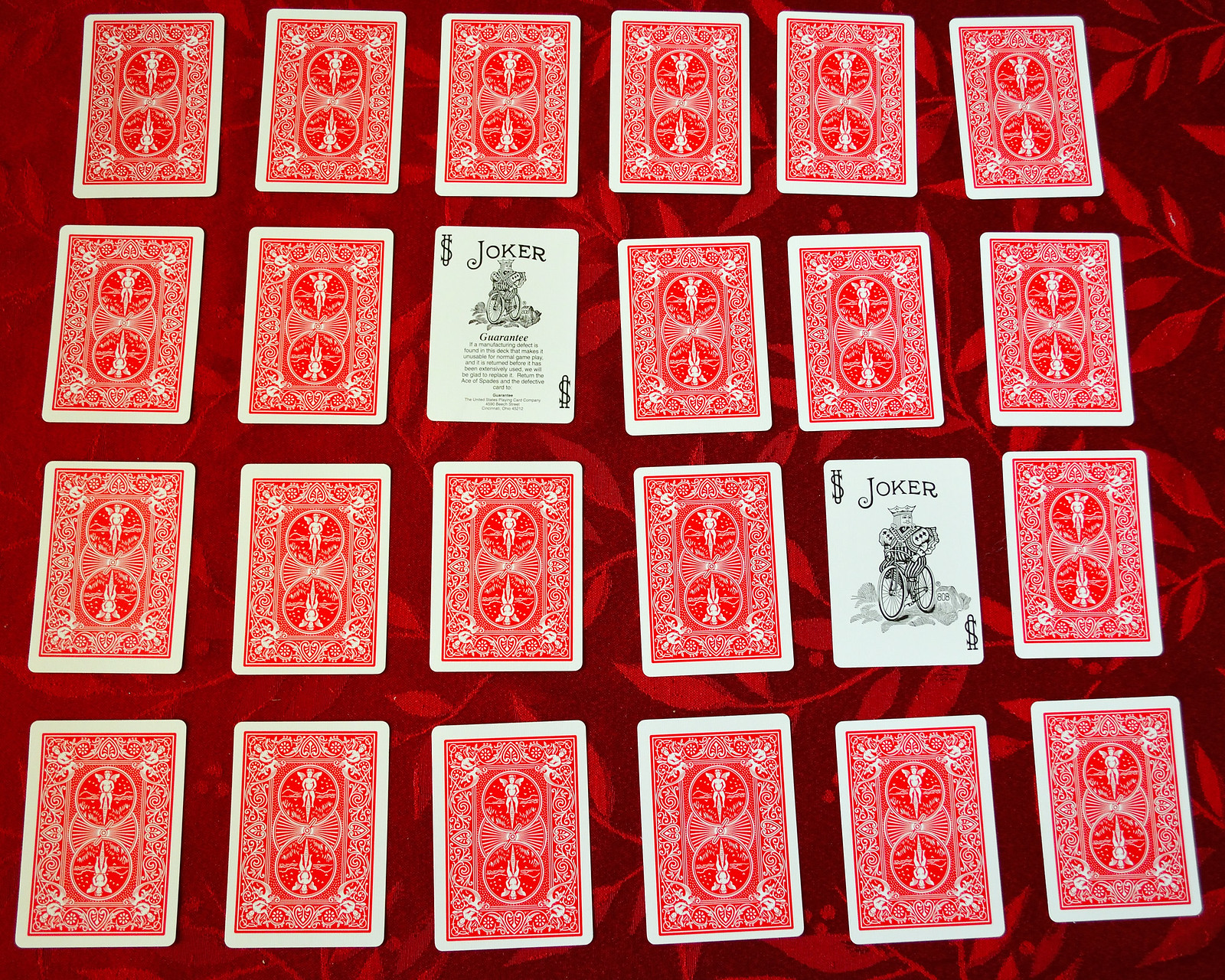This horizontal photograph captures a neatly arranged display of playing cards. All cards, except for two, are face down, revealing their red backs adorned with two interlocking circles and intricate white designs. These cards are methodically aligned in a grid of four rows, with each row containing six cards, making a total of 24 cards.

Set against a rich red fabric adorned with a delicate vine pattern, the cards' arrangement is visually striking. The only face-up cards are both Jokers. The first Joker, positioned third in the second row, prominently features the word "JOKER" in black capital letters at the top. This card also has unreadable symbols in the upper left and lower right corners, along with some text under an illustration that cannot be clearly discerned. The second face-up card, a Joker as well, is located in the third row, second card from the end. Together, these Jokers add an intriguing focal point to the meticulously structured layout of this vibrant, game-themed photograph.